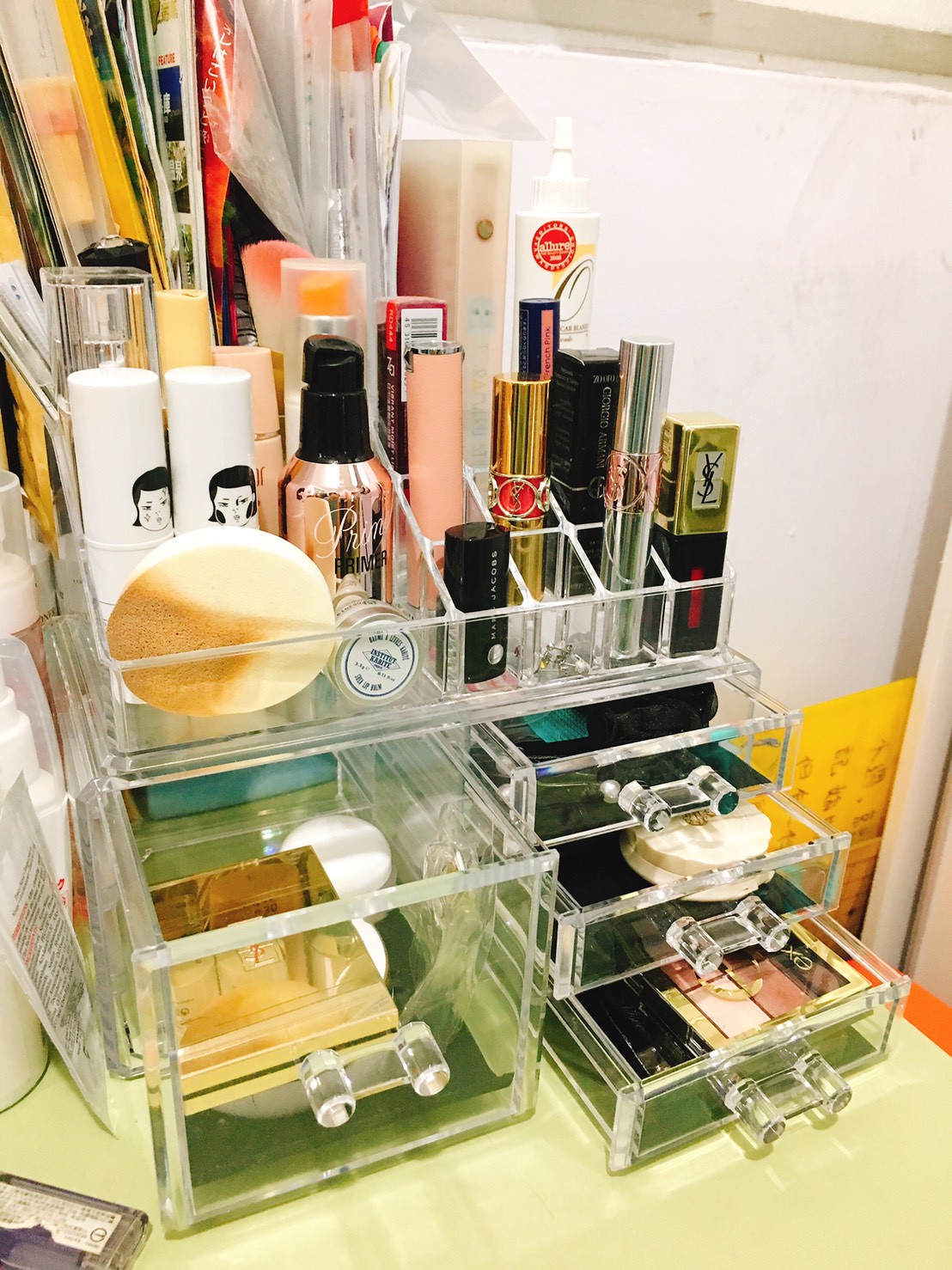This indoor photograph showcases an extensive and meticulously organized makeup collection. The collection is housed in two clear acrylic organizers stacked neatly on top of each other. The bottom organizer features a set of drawers, with a single large drawer on the left and three smaller drawers arranged vertically on the right. All the drawers are pulled out, exposing their contents. 

The large drawer on the left contains a gold compact—likely for blush or eyeshadow—and a few small white jars, presumably moisturizers, nestled underneath the compact. The right-side drawers are filled with an assortment of compacts and eyeshadow palettes. 

The top organizer holds an array of bottles and lipstick tubes. On the left side, a used white makeup sponge, marked with foundation, rests prominently. Behind it, a bottle of primer and several makeup setting sprays or skincare products occupy the space. On the right side, the collection includes various lipsticks, with at least three from the YSL brand and one from Marc Jacobs. The packaging and logos of other lipsticks remain indistinct. Among these items, a conspicuous bottle bearing an Allure magazine award shines, adding a touch of prestige to the collection. 

The overall composition highlights a well-curated makeup ensemble, underlining cleanliness and order, with each item easily visible and accessible.